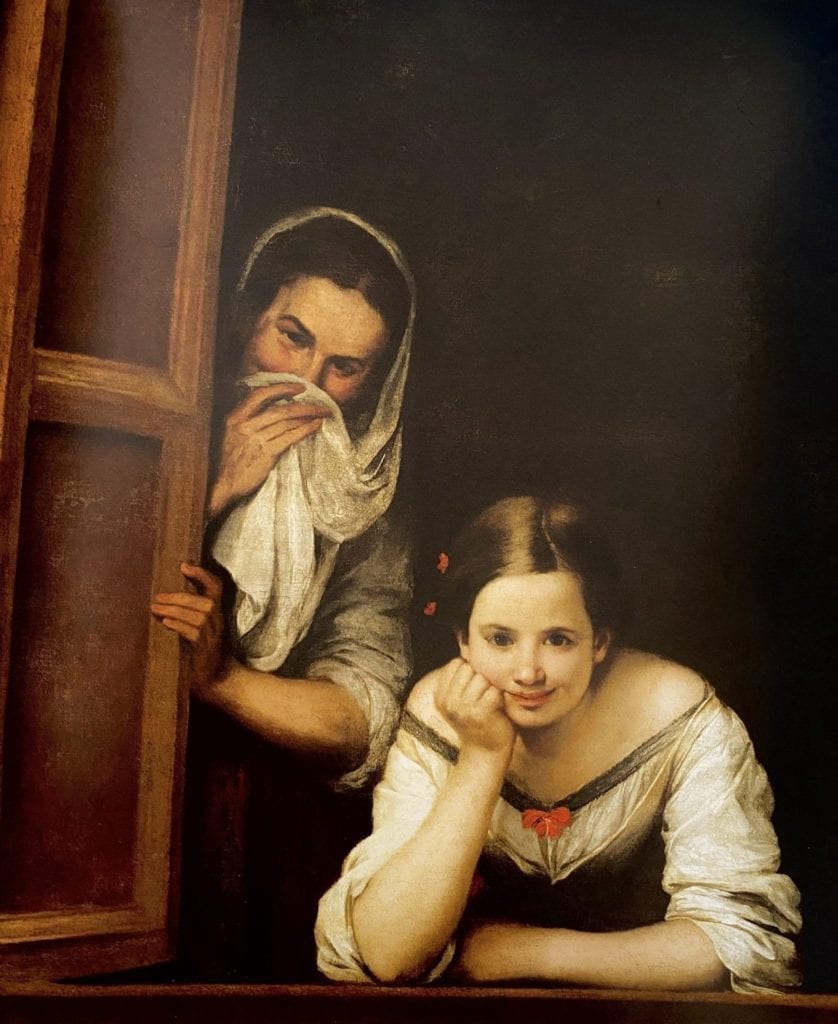This painting, evoking a vintage atmosphere, depicts two women with light complexions and brown hair looking directly at the viewer through a window. On the left stands an older woman with dark eyes and a scarf or kerchief partially covering her mouth, which she holds with her right hand, showing a hint of a smile through her expressive eyes and cheeks. With her left hand, she props open the window. The younger woman, situated on the lower right, appears to be in her late teens and is wearing a white dress that precariously hangs off her shoulders. The sleeves of her dress are rolled up, revealing her forearms. She rests her head on her right hand, her fingers curled into a loose fist, displaying a relaxed and humble demeanor. Her hair, parted on one side and pulled tight, glistens with a polished shine and is adorned with two small red flowers, complemented by a small red bow at the center of her dress. Both women exude happiness, creating an engaging and joyful scene against a stark, dark background.